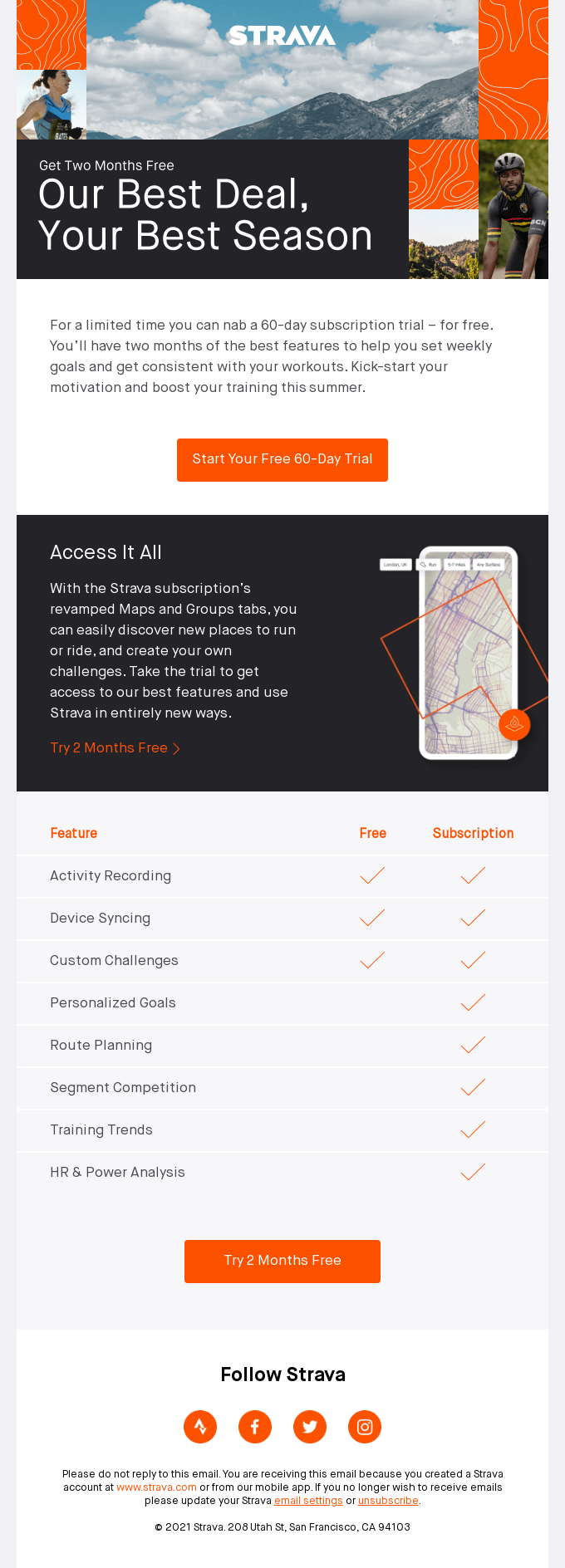The image depicts the homepage of a website named Strava. The top of the page prominently features the word "Strava" in white letters set against a picturesque background of clouds in the sky, with a mountain range faintly visible in the distance. On the left side of the header, there is a small image of a woman running, while the far right side displays a photograph of a man engaged in mountain biking.

Beneath the main title, large text reads "Our Best Deal, Your Best Season," followed by a paragraph detailing relevant information. Below this section, there is a notable black bar which includes an image of a map, resembling those found on mobile or GPS tracking devices. Further down, the page lists several items and features available in what appears to be the Strava app. Finally, an orange button near the bottom invites visitors to "Try Two Months Free."